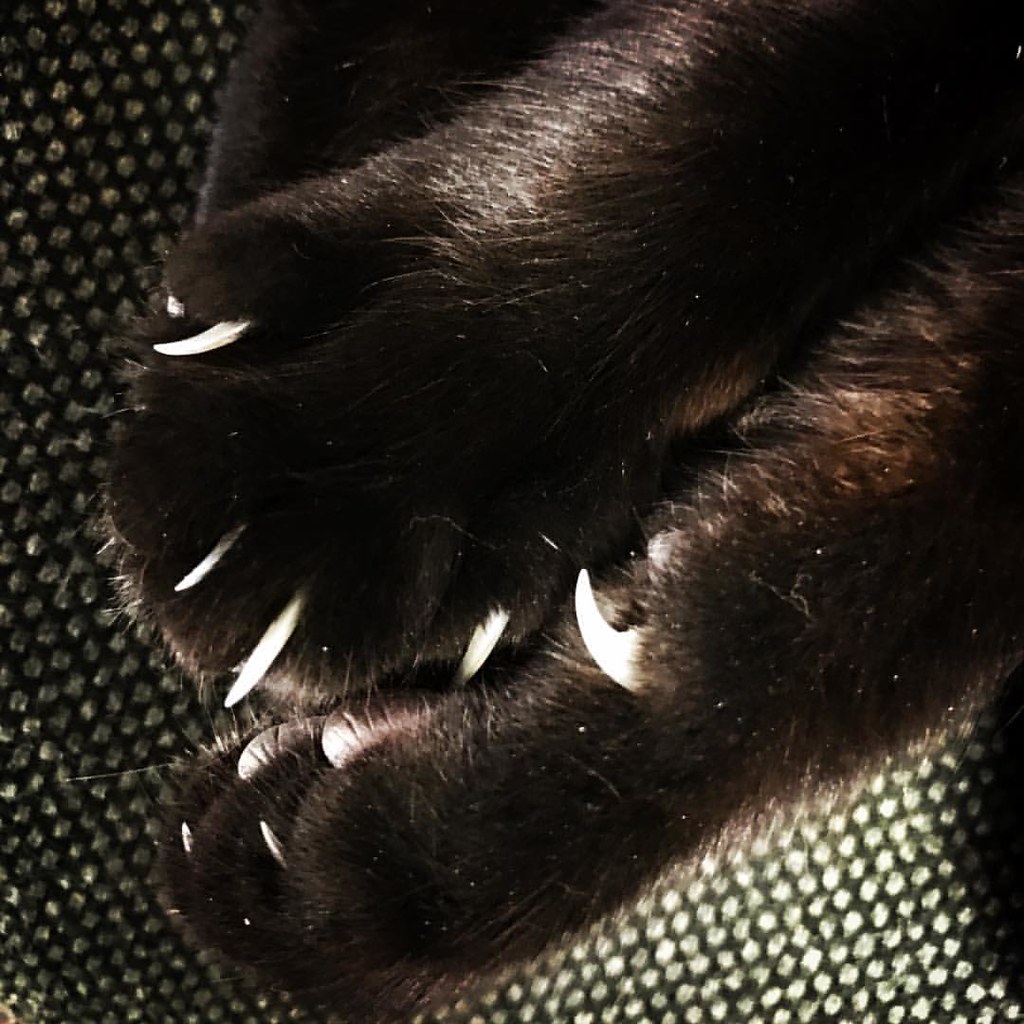This close-up photograph captures the outstretched paws of a black house cat, appearing well-groomed and healthy. The image focuses on the contrasting detail of the cat’s claws; the top paw lies almost flat with claws extended downward to the bottom left, while the bottom paw faces up towards the top left, with its claws slightly curving in that direction. The sparse hint of brown in the fur suggests it may be influenced by lighting. The surface beneath the paws is a rugged, dotted texture that resembles a metal or possibly a detailed blanket. This setting contributes to a cozy, relaxed atmosphere, indicating the cat is likely curled up and at rest. The photograph, seemingly taken while the cat was asleep, emphasizes the serene and calm demeanor of the animal.